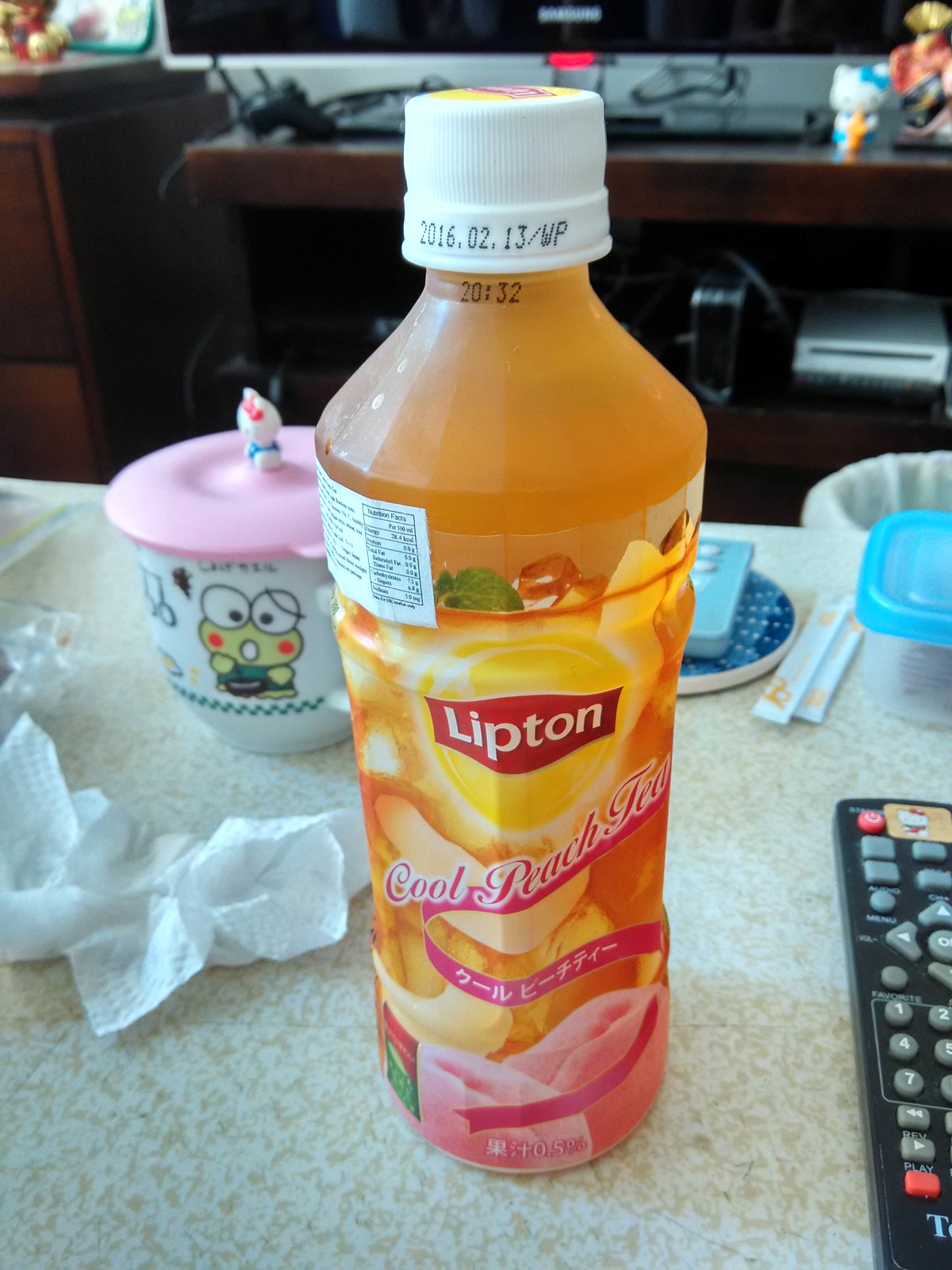On a white countertop with brown speckling sits a black remote control adorned with a yellow Hello Kitty sticker at the top. The remote has a variety of buttons including a grey button array on the left, arranged in a number pad sequence from 1 to 9. In the middle, there are directional arrow buttons pointing up, down, left, and right. Additional buttons for functions like fast forward, play, and a red stop button are also present.

To the left of the remote is a bottle labeled "Cool Peach Tea," featuring pink ribbons on its design. The bottle contains an orange liquid, with the top marked with "2016.02.13/WP" and the numbers "20" and "32." 

Behind the bottle stands a crumpled-up napkin and a pink sippy cup topped with a Sanrio character design featuring a green frog. There is also a plastic container with a blue lid nearby. In the background, a TV with a "Buzzwong" display is visible, along with various electronic devices.